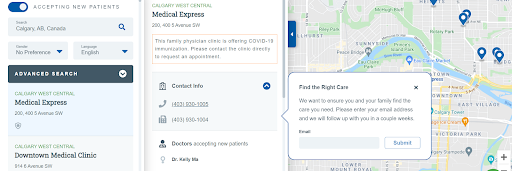In this image, we see a detailed screenshot from a medical website interface. On the left-hand side, there is a prominent toggle switch labeled "Accepting New Patients," which is turned on. Below this, a search bar displays a Canadian address, suggesting a location-based search. The search criteria shown include "No preference" for both gender and language, with English being the default language.

Further down, there are search results listed, including entries for "Advanced Search Medical Express" and "Downtown Medical Clinic." The entry for "Medical Express" is expanded, revealing more detailed information. A pop-out section to the right provides the contact details for Medical Express, including a phone number and building number, although the text is too pixelated to read clearly. Beneath this section, there is a note indicating that doctors at this facility are accepting new patients.

On the right-hand side of the image, we see a map displaying various medical locations marked with small blue pins, representing different medical facilities. Additionally, there is a pop-up message that reads "Find the right care," accompanied by a field to insert your email for further assistance or information.